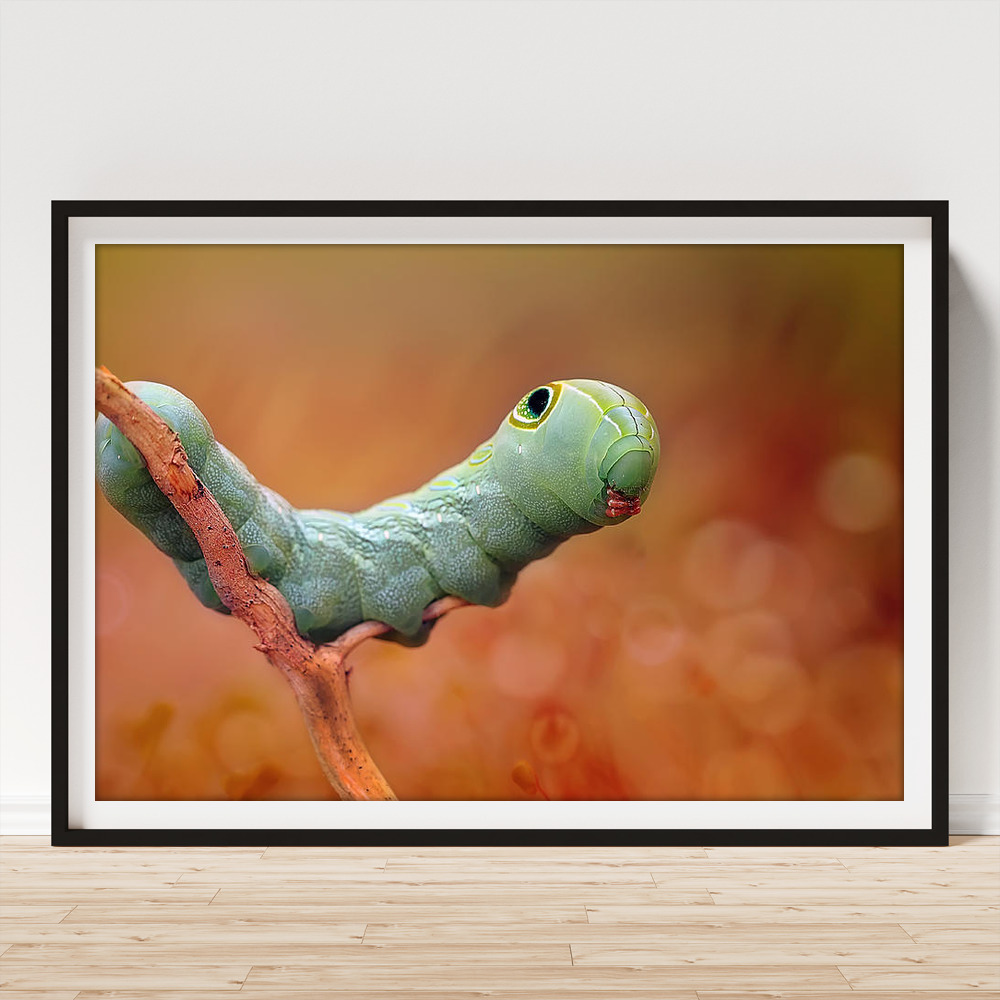This detailed image shows a large picture frame with a solid black border, set against a uniform white wall on a smooth, light-colored wooden floor with horizontal slabs. The black-framed picture includes a white border, drawing attention to the central image of a large, vividly detailed green caterpillar. The caterpillar, adorned with yellow stripes and black and green eyes outlined in yellow, is perched on a brown branch that diagonally crosses from the bottom center to the top left of the image. The caterpillar appears to be climbing sideways from left to right, with its mouth resembling a parakeet’s beak, and orange accents at its bottom. The background of this captivating close-up is a subtle, blurred mix of brown and orange hues.